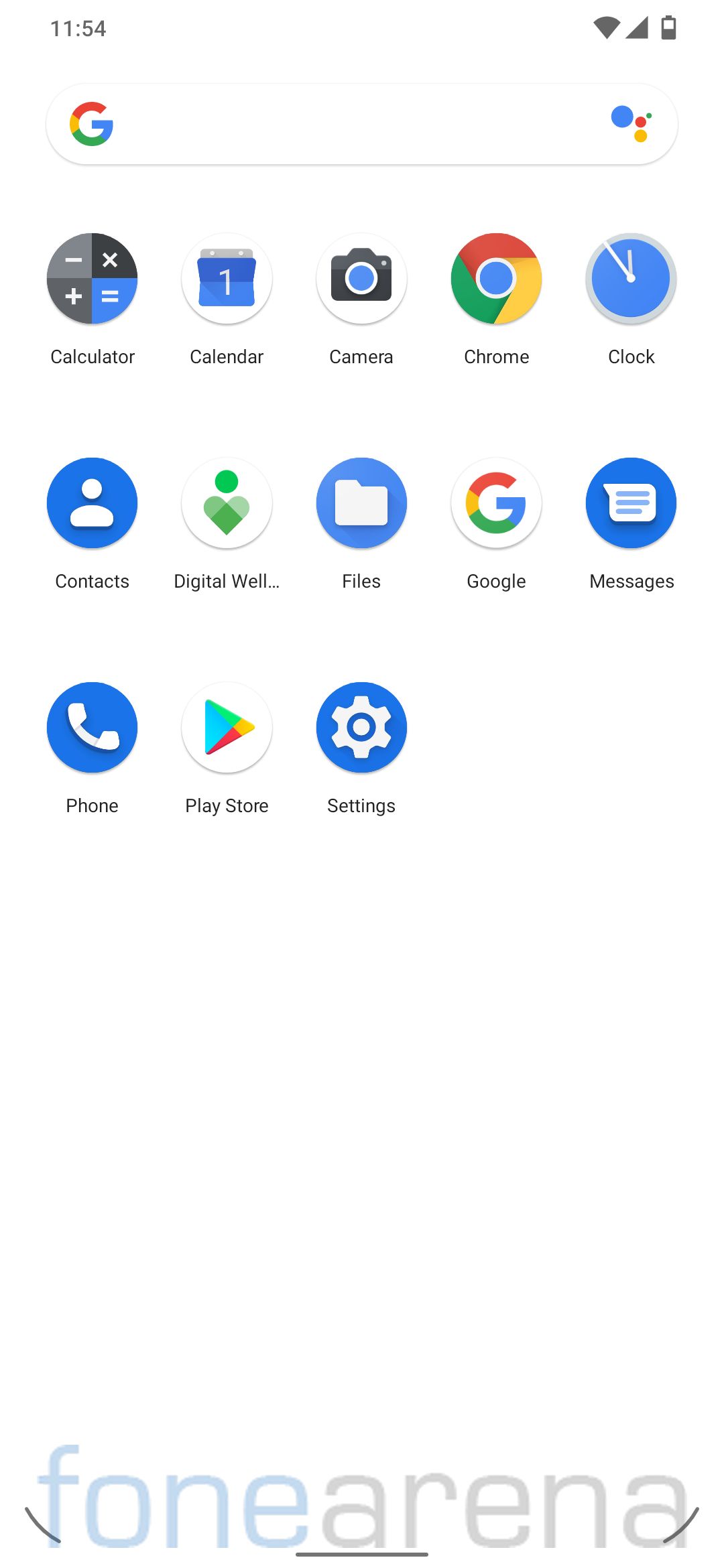This is a descriptive caption for the given image:

"A screenshot displaying the home screen of an Android phone. In the upper-left corner, the time is visible. The upper-right corner shows the Wi-Fi status. Below, a Google search bar followed by several app icons is prominently featured. The available apps include Calculator, Calendar, Camera, Chrome, Clock, Contacts, Digital Wellbeing, Files, Google Messages, Phone, Play Store, and Settings. Many of these icons are blue in color. The bottom of the screen carries a watermark with 'fone arena' in a translucent style, 'fone' being blue and 'arena' gray, with approximately 50% opacity. The bottom of the image also includes lines indicating the edge of the phone. The overall composition is a typical Android home screen with various essential apps arranged neatly."